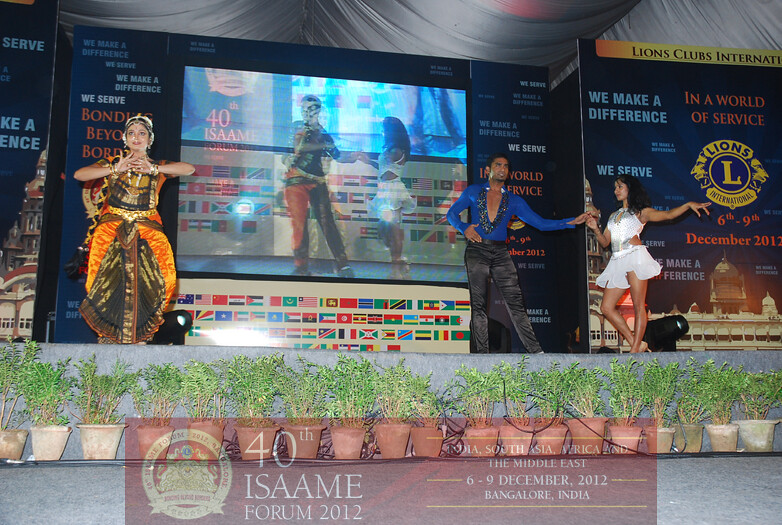The photograph shows a dynamic stage performance at the 40th ISAAME Forum 2012 held from December 6 to 9 in Bangalore, India, organized by Lions Club International. Center stage is a vivid depiction of Bollywood-style entertainment, featuring both traditional and modern dance elements. In the foreground, a woman adorned in a striking orange sari and elaborate headwear performs a traditional Hindu dance. She stands beside a couple dressed in contrasting modern attire: the male dancer in black pants and a tight blue shirt, and the female dancer in a white dress. Behind them, a large screen mirrors their lively performance, providing a magnified view of the action. Flanking the stage are banners and placards, one listing countries like India, South Asia, Africa, and the Middle East. At the bottom of the photo, a row of potted plants adds a touch of natural beauty. The setting is festive and colorful, capturing the essence of a global cultural celebration and the spirit of unity and service fostered by the Lions Club International.